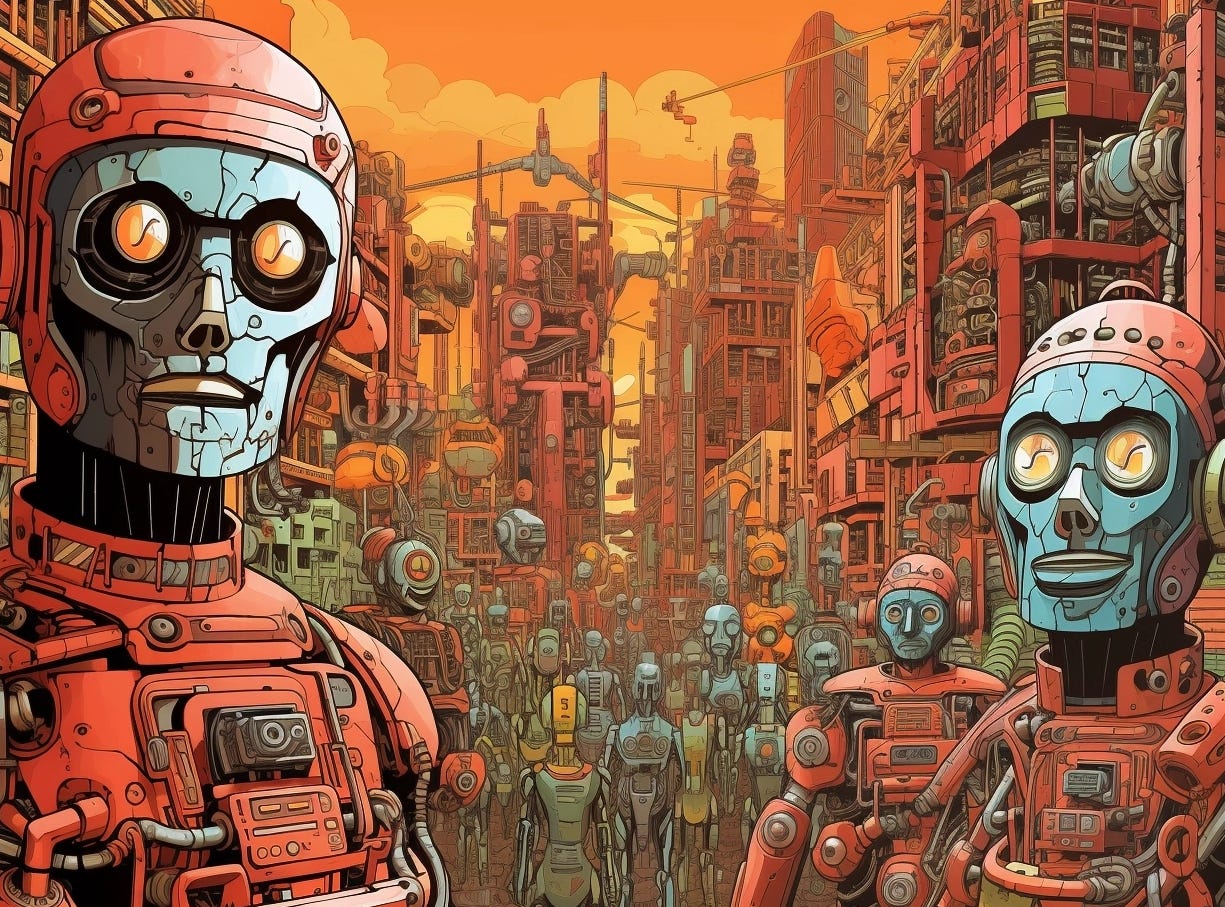In this vibrant, futuristic comic book illustration, the predominant tones of orange and red fill the large sky, accentuated by varying shades of yellow clouds. The scene showcases a sprawling, cyberpunk-inspired city with tall, complex buildings that possess an industrial, almost steampunk aesthetic, adorned with numerous gadgets and mechanical embellishments.

Prominently in the foreground are two humanoid robots with blue-grey metallic faces, glowing yellow eyes, and red helmets. Their bodies consist of intricate mechanical parts, flexible piping, and visible cables around their necks. One stands on the left, while the other is positioned on the right. A third robot, along with numerous others, is scattered throughout the city's background, all sharing a similar design but varying slightly in color, with some displaying additional blue and red hues.

The overall scene is filled with these mechanical beings, adding to the intense, almost ominous atmosphere created by the orange sky and the futuristic urban landscape. The drawing integrates muted shades, making it colorful yet cohesive, and effectively captures the essence of a technologically advanced city dominated by robotic inhabitants.